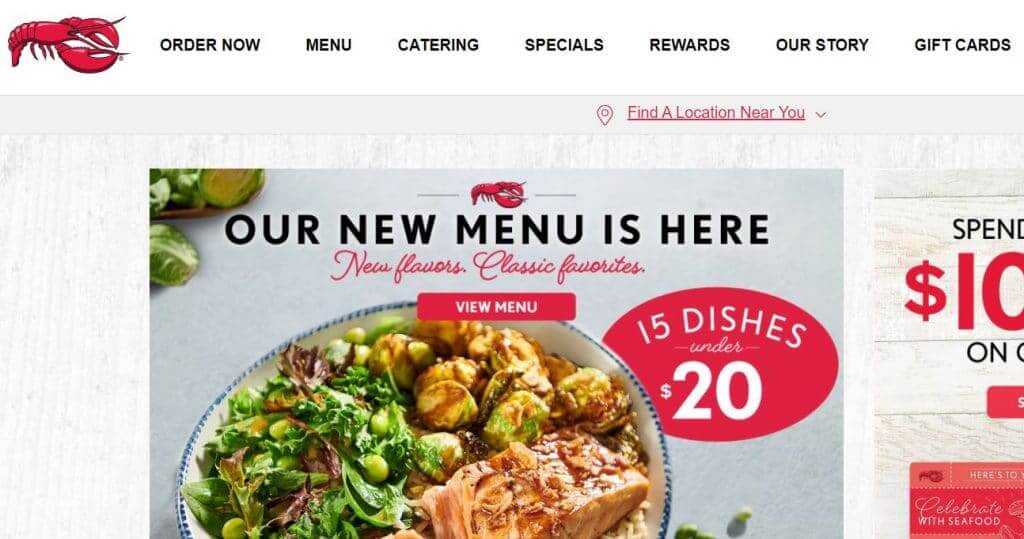This screenshot showcases the homepage of the Red Lobster restaurant website on a computer screen. The top section of the screen is white, featuring a stylized drawing of a red lobster in the top-left corner, with the tail on the left and the claws on the right. Along the top of the screen, there are several navigation options in dark black text: "Order Now", "Menu", "Catering", "Specials", "Rewards", "Our Story", and "Gift Cards".

Below the navigation menu, the screen displays a textured gray rectangular section. Centered at the top of this section in red is a location icon accompanied by a link "Find a Location Near You". Dominating the majority of the background is a vibrant picture showcasing a dish from the Red Lobster menu. Above this image, the text reads "Our New Menu is Here" in bold black letters. Beneath this, in red script, it says "New Flavors, Classic Favorites." A prominent red button with white text labeled "View Menu" is placed below this tagline.

Adjacent to the dish, there is a red oval shape containing the text "15 Dishes Under $20" in white. To the right, partially visible information seems to advertise some offer, starting with the word "Spend" in black letters, followed by "$10", and the preposition "on". Below this, a red button hints at further details, and the cut-off red information below faintly reveals the phrase "Celebrate Seafood". The partial visibility suggests more content beyond the screen's captured area.